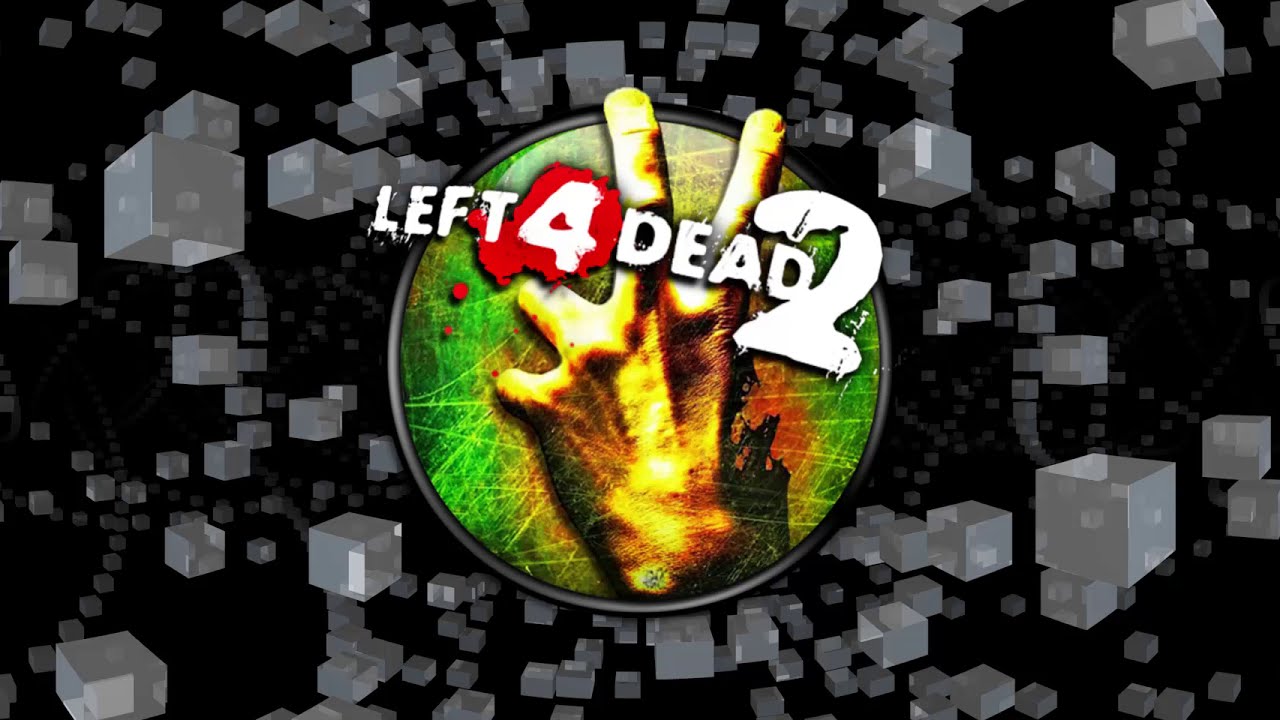This digital image features a black background adorned with an array of semi-transparent white and gray cubes of varying sizes, randomly distributed across the scene. Some cubes appear to float high on the screen, while others are at the bottom, creating a dynamic and multi-directional layout. At the center of the image is a prominent round emblem with a vibrant etched background in hues of green, yellowish, and reddish tones, simulating toxic metal with scratches. Dominating the center of the emblem is a distressed hand with a gruesome appearance, showing four fingers, with two fingers distinctly upright and colored in vibrant yellow. The hand appears gnawed off, amplifying the horror element. Overlying the emblem, in splattered white text, are the words "Left 4 Dead 2," with the number 4 prominently placed over a blood red splotch, enhancing the eerie and chaotic feel of the logo. The transparent cubes seem to curve and swirl around the central emblem, adding to the ominous and unsettling atmosphere of the composition.